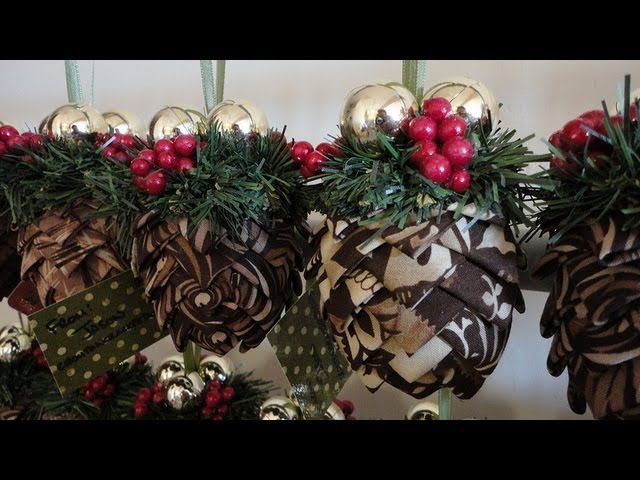This photograph captures a series of intricately designed Christmas decorations hanging against a white background. Each ornament resembles a pinecone, crafted from brown and white cloth folded into a textured, organic shape. Atop the cloth base, there is a festive arrangement of artificial green foliage, mimicking holly, adorned with clusters of bright red berries. Adding to the sparkle, silver balls crown each pinecone ornament, with reflections of the photographer visible in their shiny surfaces. Attached to the ornaments are loops of green twine for easy hanging, suggesting their use as tree decorations. Additionally, a green tag inscribed with "from Jason" is visible among the decorations. The ornaments are suspended close to one another and appear to be connected by their green ribbons, creating a harmonious and elegant display.